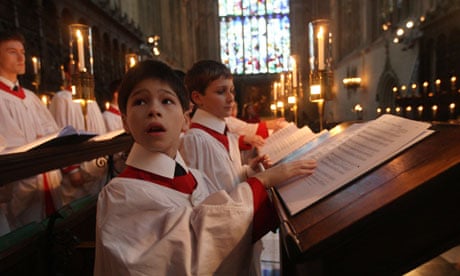The image captures a small group of choir boys singing inside a Catholic cathedral. They are dressed in white cassocks with red shirts and stiff white collars, giving them a formal appearance reminiscent of a public school uniform. In the foreground, a wooden slanted music stand holds their white music books, though the notes on the pages remain unreadable. Most of the children are intently focused on their music, except for the boy at the front who has turned his head, looking slightly surprised or shocked, possibly at the camera. The background features a softly lit stained glass window and numerous candles in gold-colored holders, framing the serene and solemn atmosphere of the scene. The choir boys, with their dark hair and solemn concentration, are bathed in the gentle, colorful light filtering through the stained glass, highlighting the sacredness of the moment.